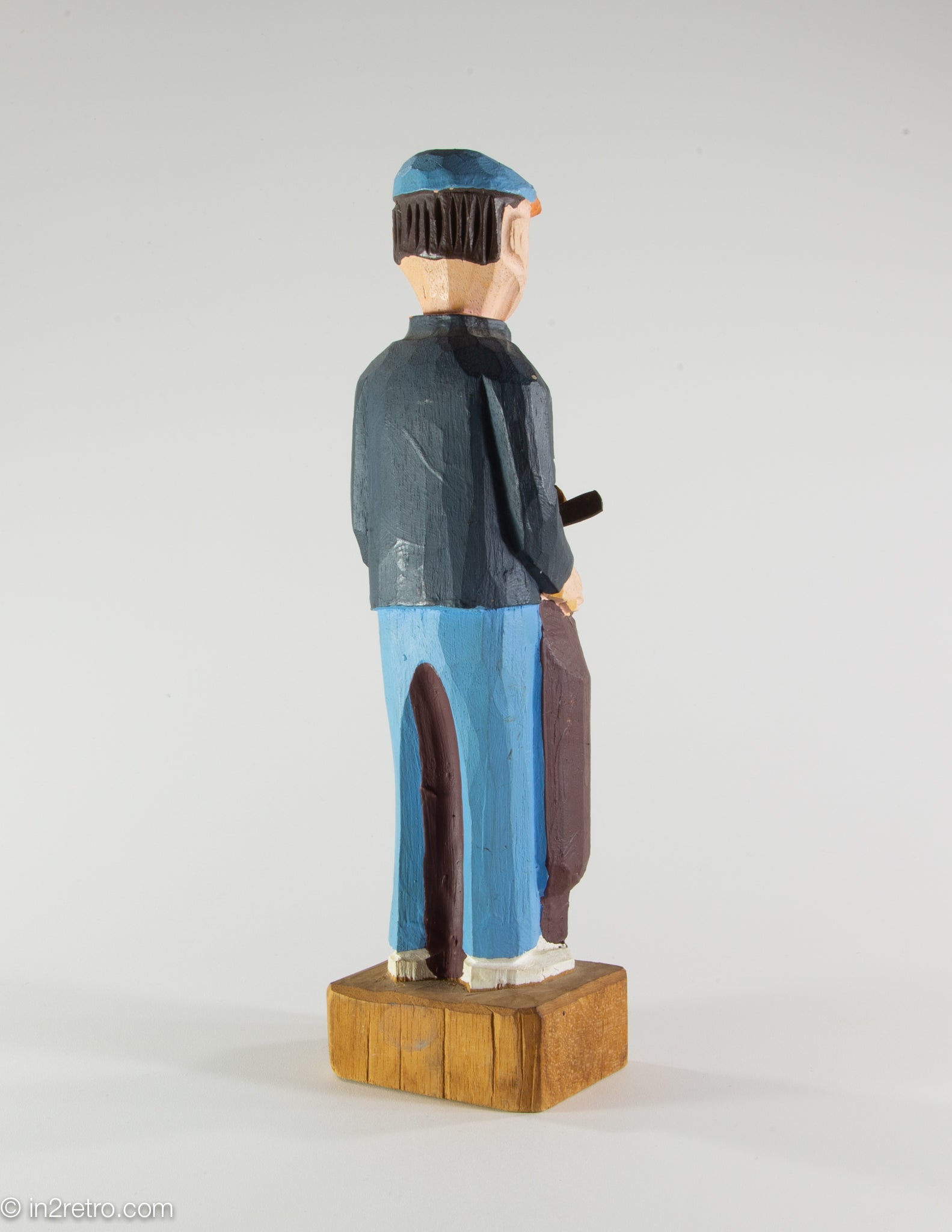This detailed wooden sculpture showcases the back of a man meticulously carved from wood and painted. He stands on a small wooden base, adorned in blue pants and white shoes. The man is clad in a darker blue jacket, potentially mixed with grey hues, and a matching blue newsboy cap. His hair is intricately carved to simulate strands, and his light skin accents his dark hair. Notably, his carved ear and the brim of his cap are visible. The man is holding what appears to be a bag, with something dark, possibly black, protruding from it, suggesting he could be a golfer holding a golf bag. The sculpture is displayed against an off-white background, and at the bottom left corner, there is a copyright mark: “I-N-2-R-E-T-R-O dot C-O-M.”